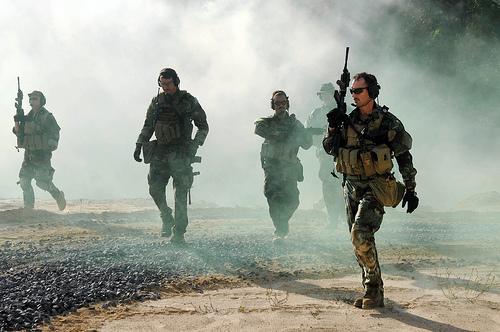In this detailed image, five soldiers are seen walking through a thick, dense cloud of white and light gray smoke, emerging dramatically onto a gravel path mixed with patches of light-colored sand. Their shadows stretch prominently to the right under the bright sunlight that pierces through the smoky haze. All soldiers are dressed in camouflage Army fatigues, with gear strapped around their waists and torsos, and they all sport combat boots. The soldier at the forefront on the right is particularly noticeable; he wears sunglasses and a headset with a microphone, and he holds an automatic rifle pointed upward close to his body. To his left, another soldier is holding his gun high in the air. Among the group, most soldiers have headgear, with one clearly displaying a radio headset. One soldier, partially obscured by the smoke, trails behind, making his features less distinguishable. As they march forward, their presence is striking against the backdrop of the battlefield shrouded in a swirling mist of smoke.